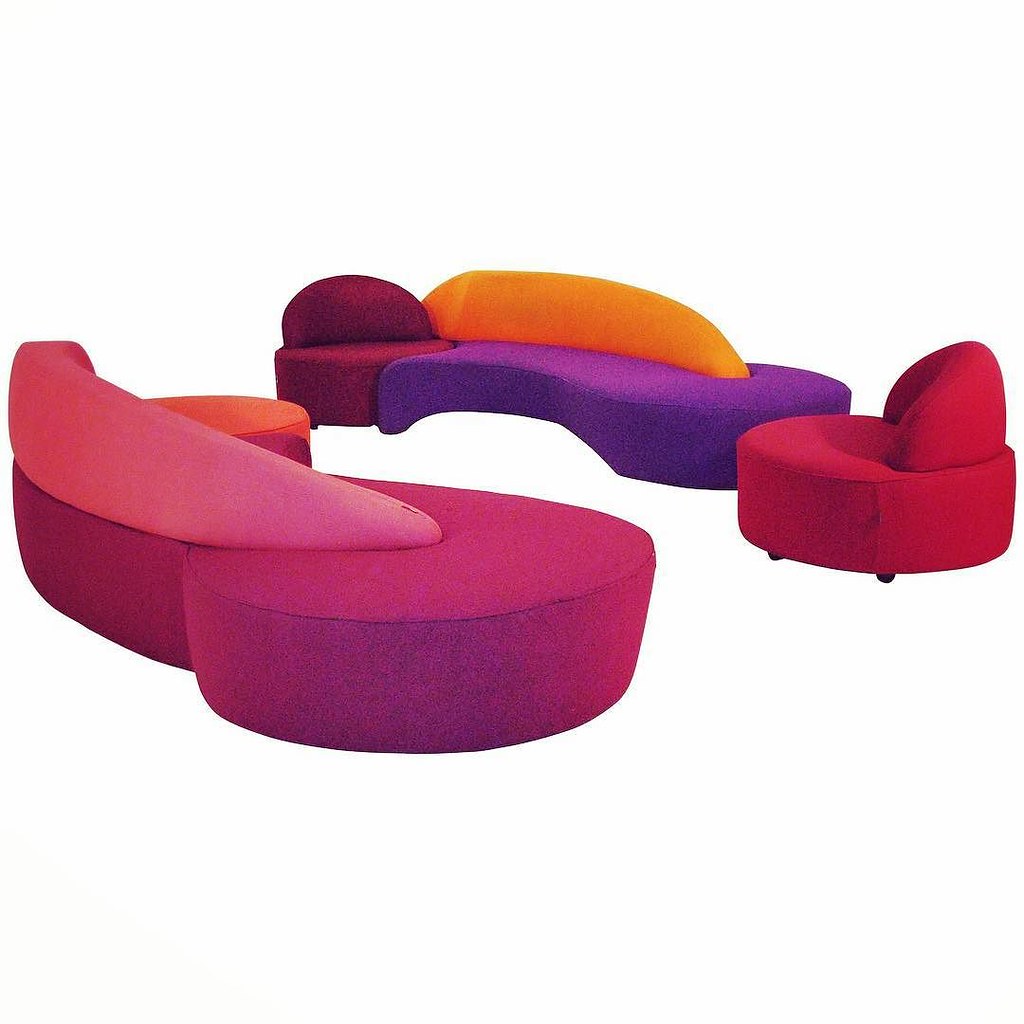This image showcases an artistic and vivid illustration of three pieces of modern furniture set against a stark white background, giving it a clean and minimalist look. The main items depicted are two sectional couches and a round chair, all upholstered in bright, eye-catching colors. The first couch, positioned at the back, boasts a primary color of vibrant purple, complemented by an orange backrest and a maroon pillow. Opposite this, the second couch features a rich magenta hue with a pink backing and a medium orange armrest. To the right of the purple sofa, there's a rounded side chair with a tubular design and wheels, adorned in a deep magenta color with a soft, cushioned back. The fluffy, unconventional shapes and the striking palette of magenta, pink, orange, dark red, light orange, and purple lend the furniture a whimsical and somewhat surreal appearance, making it resemble elements from a digital art piece or a stylized movie set rather than real-life furniture.